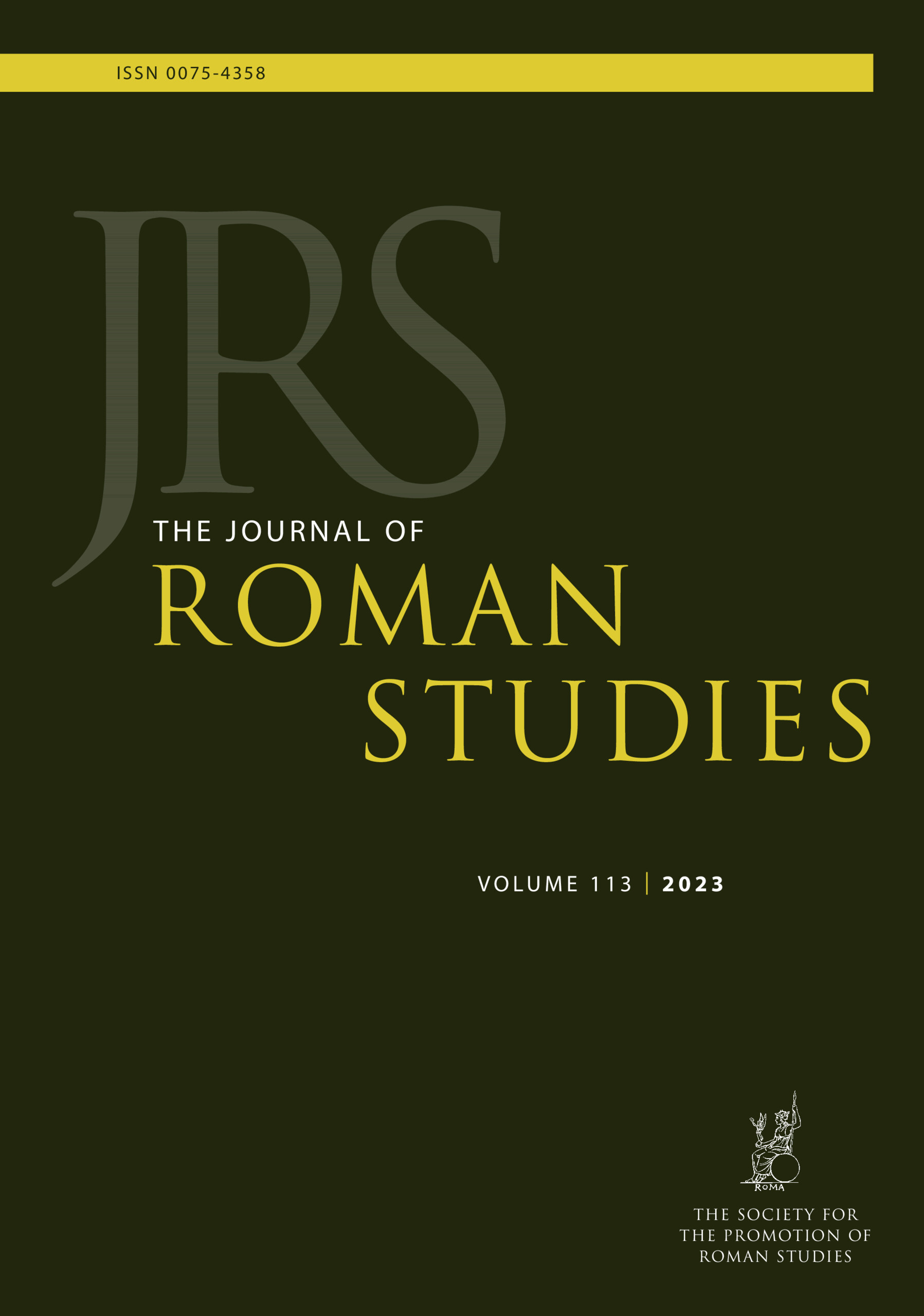The cover of the Journal of Roman Studies (JRS), volume 113, 2023, is presented in a dark olive green shade. Prominently across the top of the cover is a long, narrow, bright yellow strip containing the ISSN number 0075-4358 in black text. The title "JRS" appears in large pale gray letters, with "The Journal of Roman Studies" written beneath in white and yellow text respectively. At the bottom right corner of the cover, there is a small image that likely depicts a Roman warrior, accompanied by the text "The Society for the Promotion of Roman Studies" in white. The overall design includes accents in white and yellow that contrast against the dark olive background.